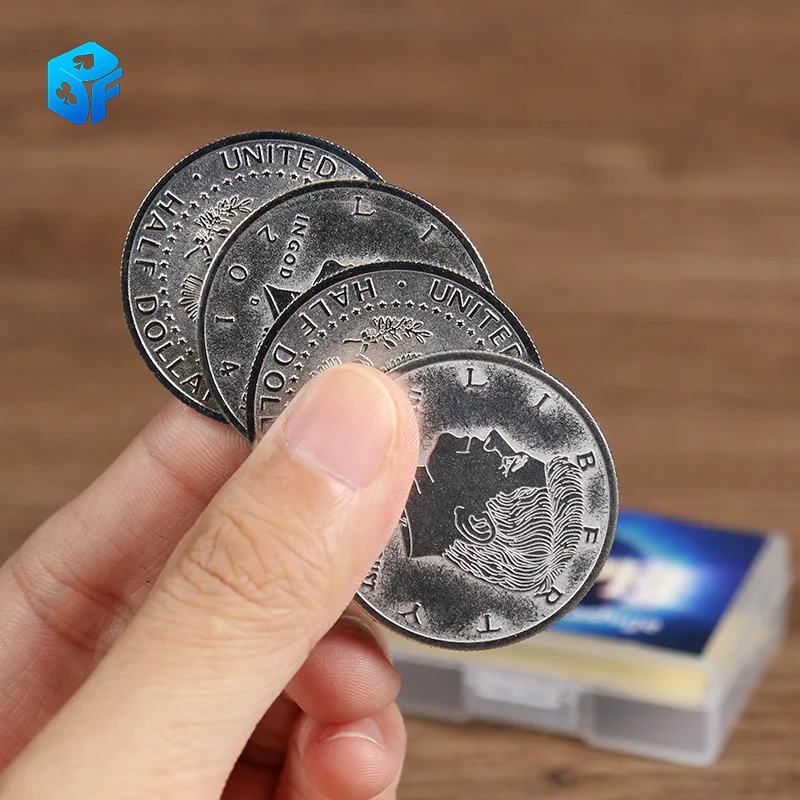This square photograph captures a close-up of a left hand, appearing to be that of a Caucasian male, holding four overlapping U.S. half-dollar coins between the thumb and forefinger. The thumb, which is at the top of the coins and is visible with a short thumbnail, emanates from the lower left corner of the image. The pointer finger is visible behind the thumb, while the remaining fingers are curled underneath the coins, their nails slightly peeking out.

The coins, arranged diagonally from the upper left to the lower right, alternate between heads and tails. The bottom right coin, which partially shows the face of JFK and the word "Liberty," is followed by a coin displaying the reverse side with parts of the words "half dollar" and "united" visible. The next coin shows JFK's profile, dated 2014, with "In God" from the motto "In God We Trust" visible. The top left coin, partially obscured by the others, shows the words "half dollar" and "united" with the "R" cut off.

The coins appear to have been altered, possibly spray-painted black with white outlines, giving them an unusual appearance. The background features an out-of-focus brown wooden surface, likely a table or plank flooring, with a blue and clear plastic container in the bottom right corner. In the upper left corner, a logo with "BF" and symbols of a spade and a club appears, potentially indicative of a brand or business.